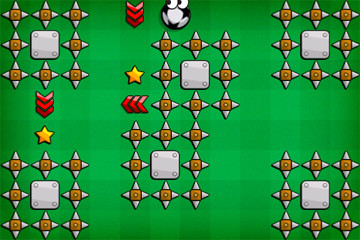This image appears to be a screenshot from a video game. It displays a green square with a checkered pattern of alternating darker and lighter green squares. Scattered across this patterned background are ninja star shapes arranged in a 3x3 grid. The center of each star features a burnt orange square. Below the main section, there are five additional sets of these 3x3 ninja star grids.

In the upper left of the image, there are three red arrows pointing downward towards a yellow star. Another set of three red arrows, located in the image's center, points to the left towards another star positioned above them. At the top of the frame, three more red arrows point directly downward. Adjacent to these downward-pointing arrows, there is a character resembling a soccer ball with large, expressive eyes looking towards the left.